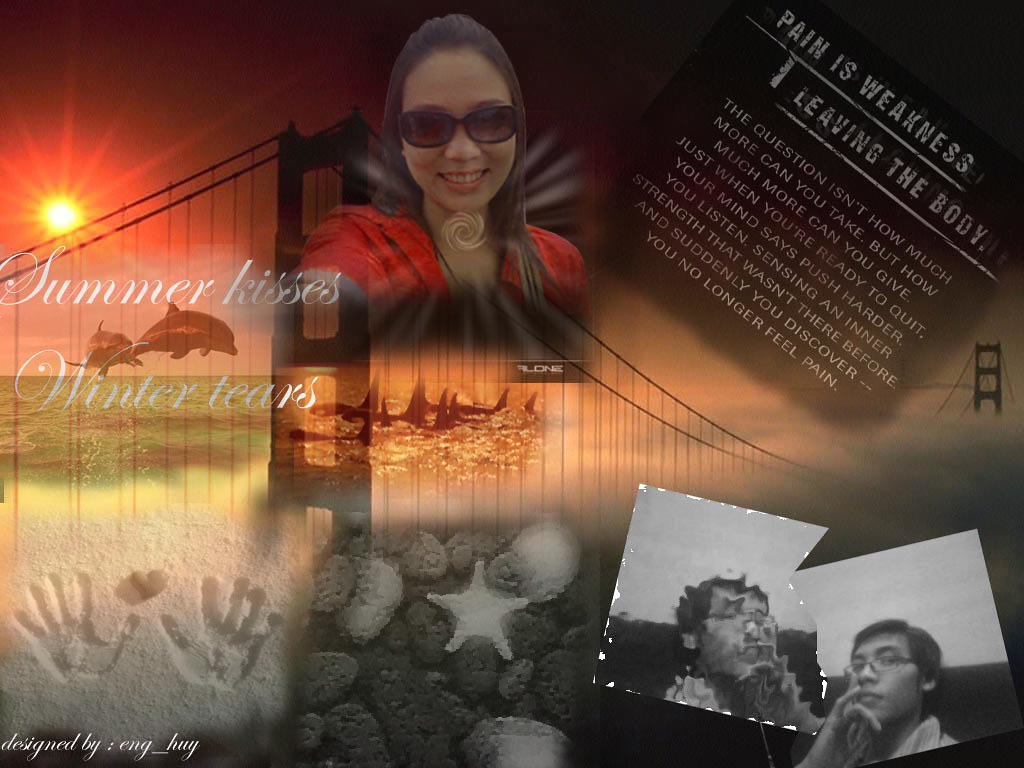The image is a wide rectangular collage featuring multiple elements. The background showcases a large bridge stretching from left to right, with two tall points—one near the left end and the other in the distant right. Beneath the bridge, a body of water hosts several dolphins leaping into the air on the left side. A bright yellow sun with long, radiant beams occupies the top left corner, casting a warm glow. Superimposed near the top center is an image of an Asian woman sporting sunglasses and a red shirt, smiling amidst beams of light. In the bottom left corner, there is an image of sand with two handprints and a heart-shaped rock nestled between them. The bottom right corner contains two images of a man, one of which is distorted and blurry. Above these elements, a paragraph of white text adorns the top right portion of the collage, alongside the phrases "summer kisses, winter tears" written near the sun and "pain is weakness leaving the body" diagonally placed. The vibrant and detailed composition captures a moment of juxtaposed themes and imagery, blending natural scenes with human elements.